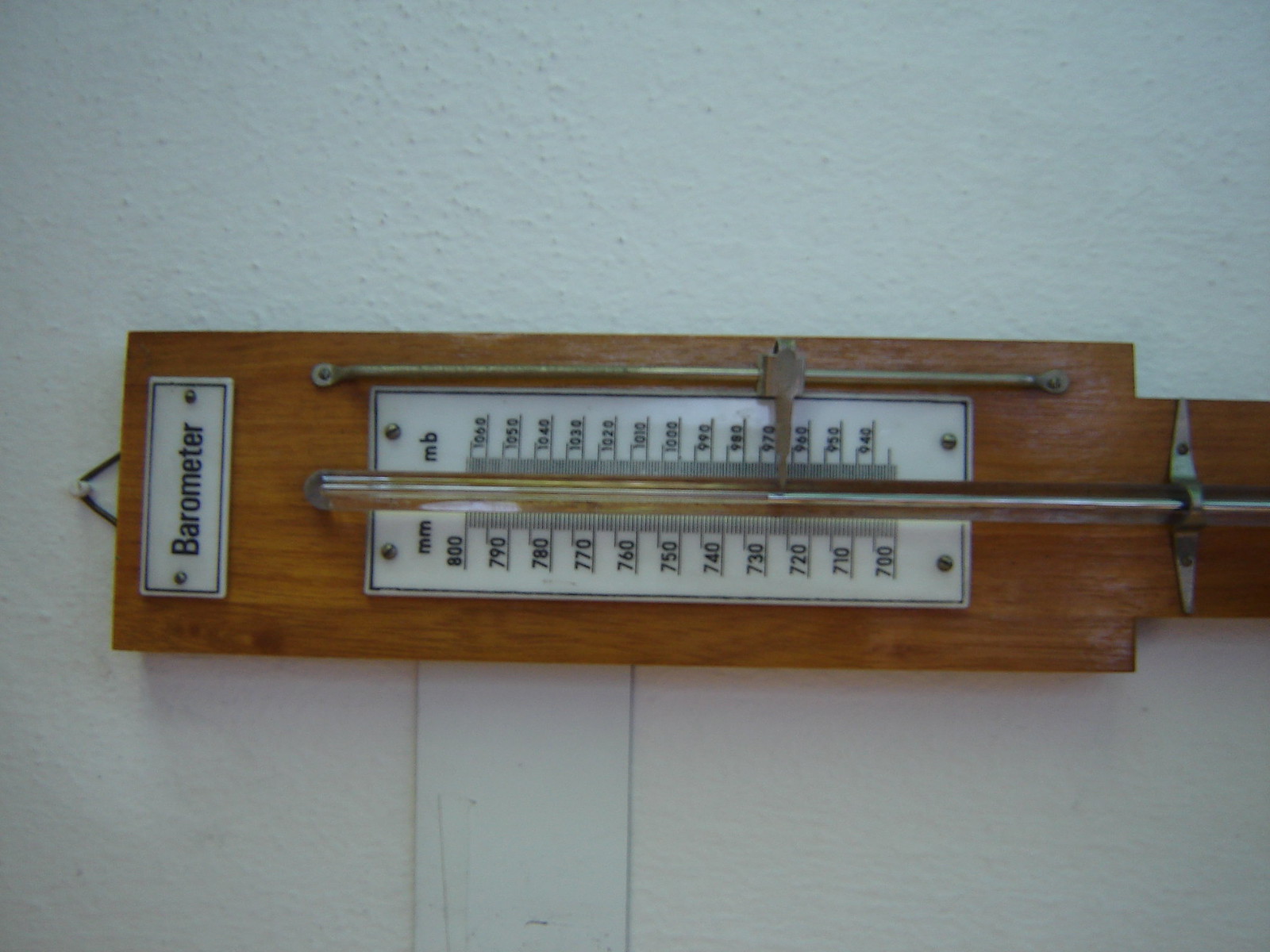This horizontal rectangular image showcases a vintage barometer mounted on a white, slightly textured wall. The barometer is encased in a wooden frame with a natural grain that is subtly glossy. Toward the ends of the wooden frame, the sides indent slightly before continuing downwards, resembling a handle; this handle-like feature is cut off midway on the right side.

On the left side of the barometer, a small white rectangular plaque hangs vertically, held in place by two screws. The word "barometer" is printed in black font on this plaque, which is bordered with a black frame and has a thin white edge protruding beyond it. The barometer itself is suspended from a small black hook attached to a peg in the wall.

Extending down from near the top of the barometer is a metal bar. The center of the barometer features a horizontal white rectangular panel secured with four screws—two at the top and two at the bottom. This panel displays the letters "MM" and "MB" in lowercase black font, written sideways, so they read correctly when viewed from the right-hand side.

The barometer includes a scale of vertical numbers running down the side on the left, starting from 800 and decreasing by tens down to 700, each number marked by longer lines protruding vertically from a baseline. Between these numbers, shorter lines denote smaller increments. In the middle, a clear glass tube resembling a thermometer is secured by a metal vertical bolt. This tube is likely used for measuring atmospheric pressure. Although the numbers on the right-hand scale are somewhat blurred and hard to read, they mirror the detailed precision of the left side.

Below the barometer, slightly off-center to the left, a white vertical plate is visible, adding to the overall composition of the wall. The wall itself is slightly textured with visible spackle, adding a touch of rustic charm to the setting in which this classic weather instrument is displayed.